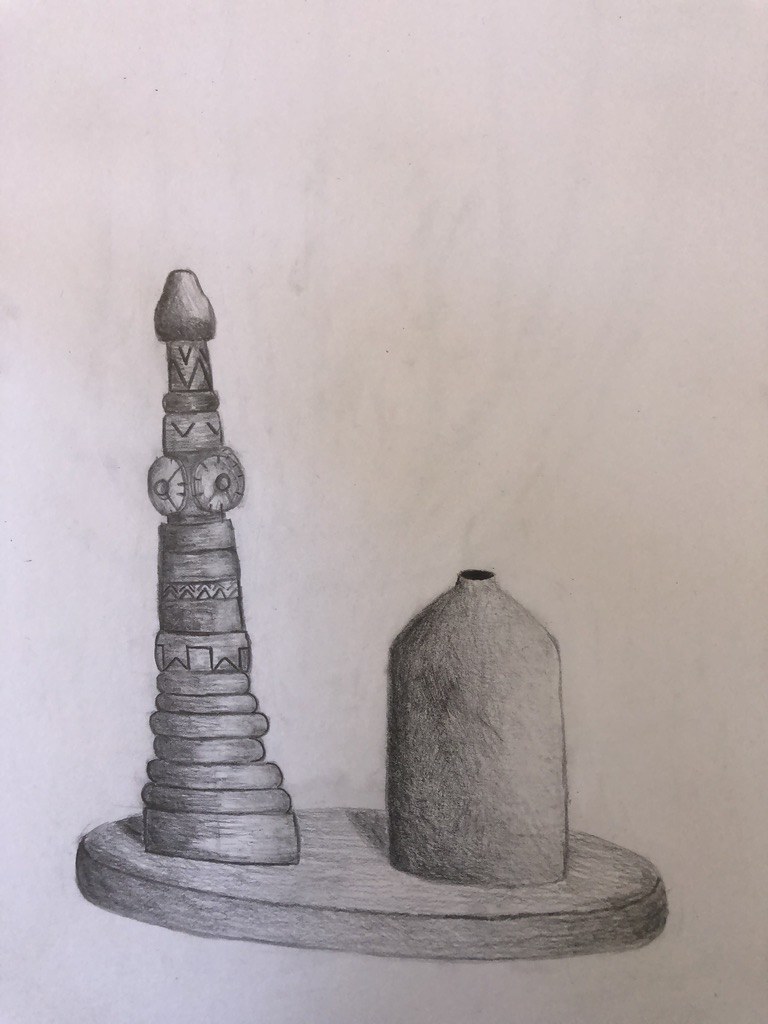This image showcases a detailed amateur art drawing set against a white background. In the composition, we see a tray on a table. On the right side of the tray, there is a jug. The top left corner is dominated by a mound of toys stacked together. The bottom right features a vase, while the left side presents a tower. At the bottom, there is a wooden disc, adding texture and contrast to the drawing. Subtle shading beneath these elements adds depth to the artwork, enhancing its intricate yet simplistic charm.